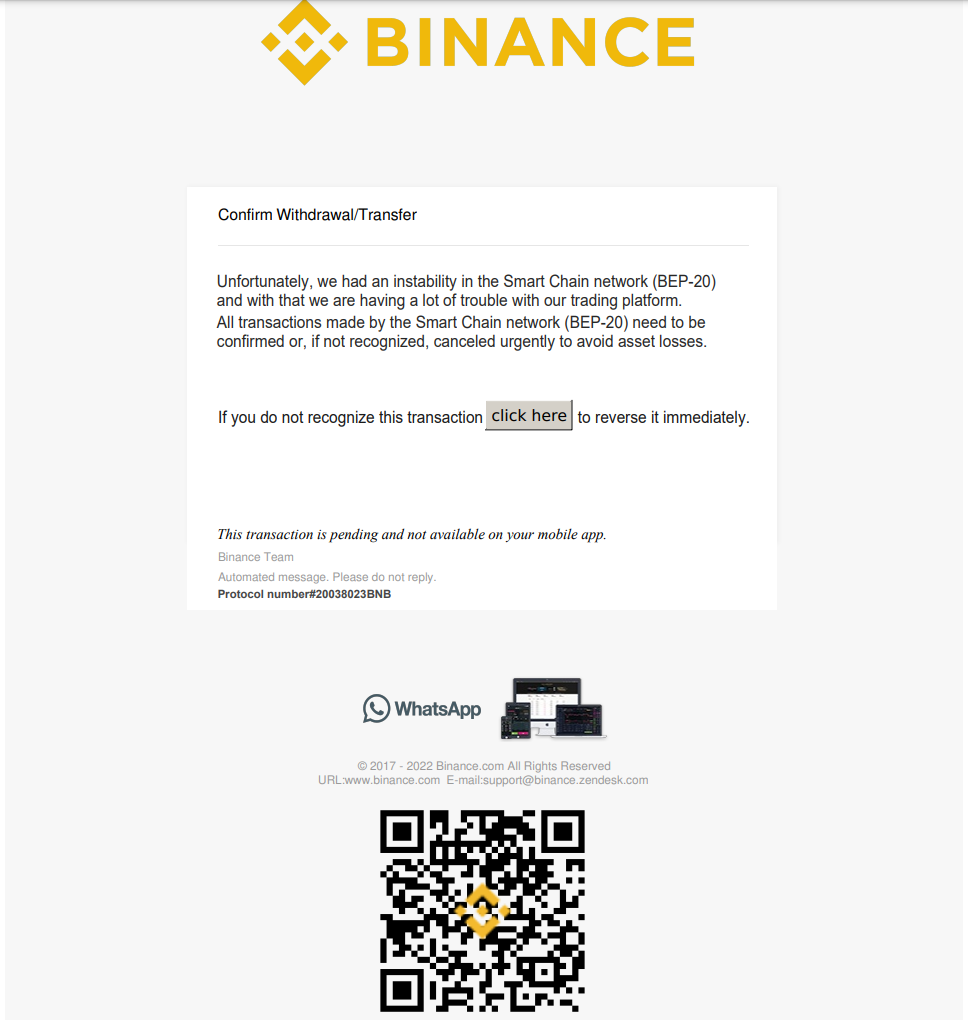Screenshot of an error message from Binance. At the top of the image, there is the Binance logo on the left and the word "Binance" in large yellow text. Two arrows, one pointing upward and one downward, are present with a diamond-like symbol in the center. The main content of the screenshot is an error message indicating issues with the Binance Smart Chain network (BEP-20). The message reads:

“Confirm Withdraw Transfer. Unfortunately, we had an instability in the Smart Chain network BEP-20 and we are experiencing significant troubles with our trading platform. All transactions made by the Smart Chain network BEP-20 need to be confirmed or, if not recognized, canceled urgently to avoid asset loss. If you do not recognize this transaction, click here.”

Beneath this, a large gray button labeled "Reverse it immediately" is visible. The alert also states: "This transaction is pending and not available on your mobile app. From the Binance team. This is an automated message, please do not reply." At the very bottom, there are icons representing WhatsApp, a laptop, and various devices, indicating the platforms through which Binance can be accessed.